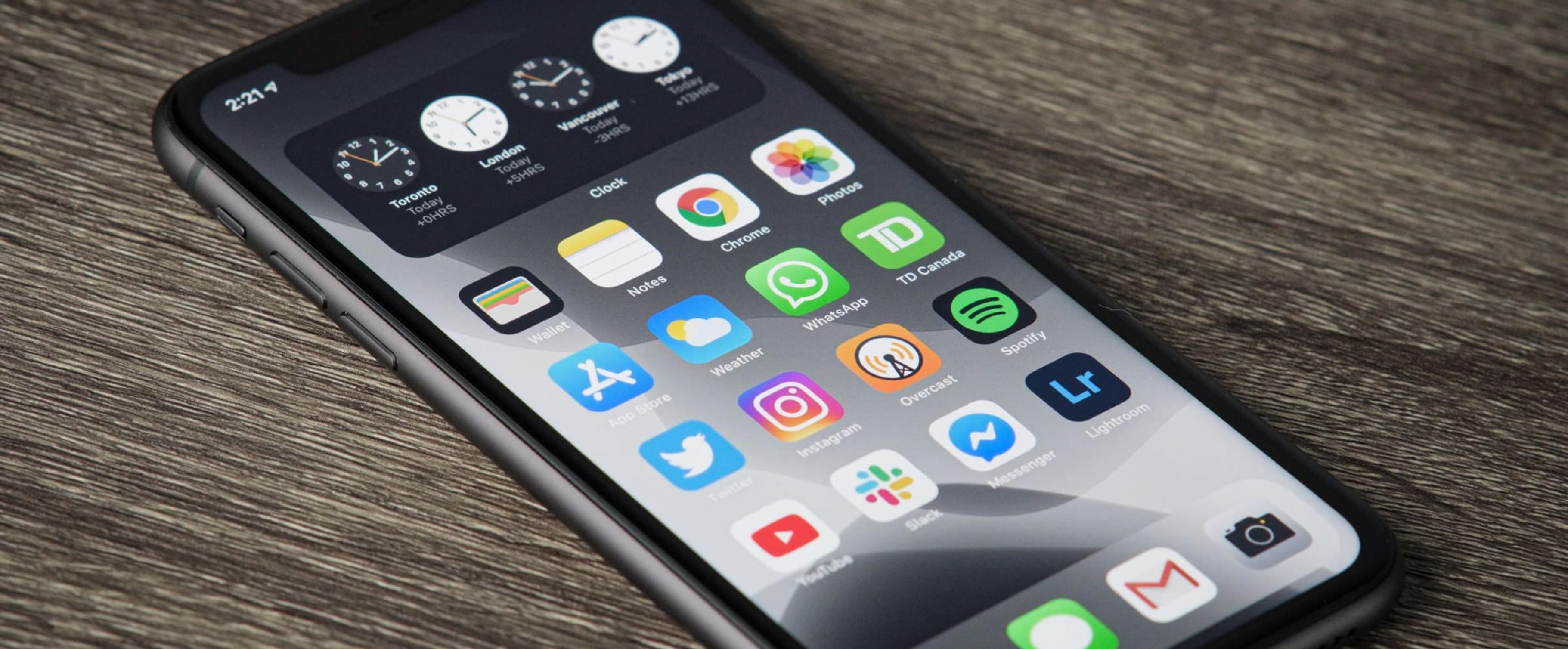This image captures a close-up of a person's cellphone, set against a grayish-brown wood grain tabletop. The phone's screen is active, displaying a clean, digitally-rendered interface that almost seems surreal in its high-definition realism. At the top of the screen, four world clocks display the current times in Toronto, London, Vancouver, and Tokyo, respectively. The device's local time, shown in the upper corner, reads 2:21.

The cellphone's home screen is organized into four rows of app icons. The first row features Wallet, Notes, Chrome, and Photos. The second row consists of the App Store, Weather, WhatsApp, and TD Canada. The third row displays icons for Twitter, Instagram, Overcast, and Spotify. The fourth and final row includes YouTube, an unreadable app icon, Messenger, and LR.

At the very bottom of the screen, there's a static dock with a text message icon labeled 'M' for email, and a camera button. The overall setup of the screen is neat and methodical, providing a glimpse into the user's organizational preferences. The sophisticated design of the phone, juxtaposed with the natural texture of the wooden table, creates a visually appealing contrast that further emphasizes the advanced technology in use.